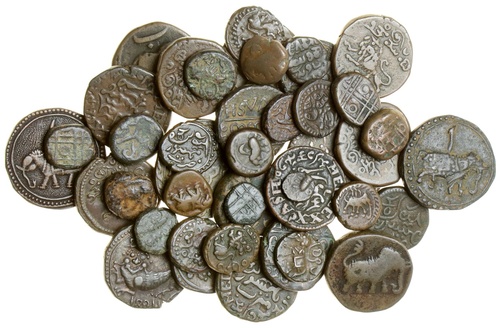The photograph displays a substantial collection of ancient coins, likely of varying origins. These coins are arranged in a pile against a stark white background, emphasizing their distinct features. They appear worn and aged, suggesting they have been in circulation for a considerable period. The majority of the coins range in color from brownish hues to silver, with some showing shades of light green and tan. The coins vary in material and thickness, with many showing signs of damage such as chipping. The designs on the coins include images of buffaloes, elephants, and lions, along with foreign scripts and markings. While their exact historical and geographical origins remain unclear, the coins' handmade appearance and diverse engravings hint at their rich and varied past, possibly from various ancient civilizations. This detailed and close-up presentation of the coins suggests they may be part of a museum collection or archaeological exhibit, focusing solely on the artifacts without any contextual background.